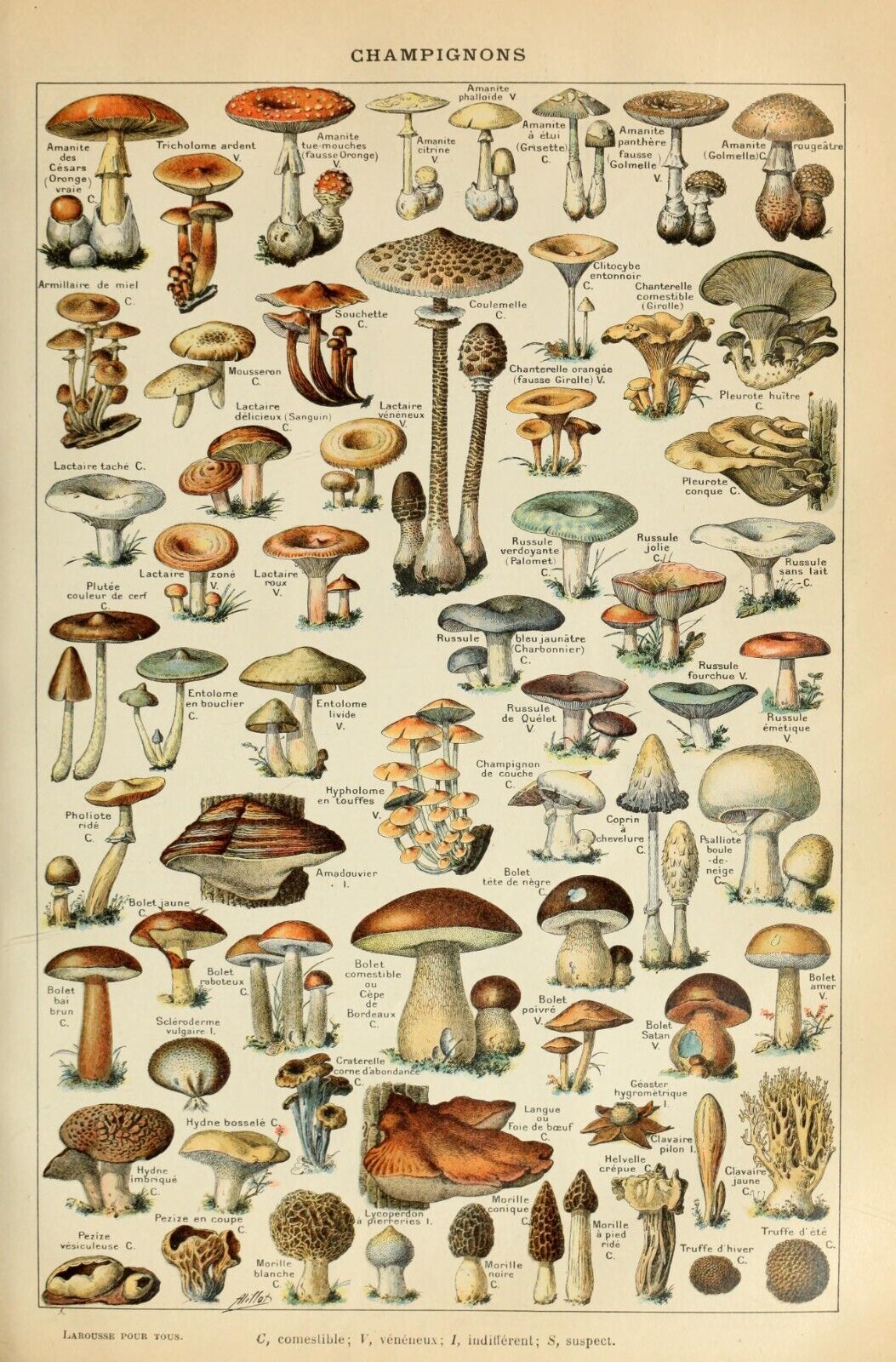This image is a detailed poster featuring a diverse collection of mushrooms on a predominantly white background, framed with a thin black line. At the top, the word "Champignons" is printed in bold black lettering. The poster showcases dozens of mushrooms, each meticulously illustrated in color, making it easier to identify various types. The mushrooms are organized somewhat randomly across the page but are all oriented upright. They vary greatly in shape and size, including some that are tiny and others that are large and take up more space. The illustrations highlight mushrooms with different colored caps, such as red and brown, and include iconic varieties like the Amanita mushroom with its distinctive red cap and white spots. Many mushrooms are depicted with small black text labels identifying them. Some are shown growing in clusters, while others appear individually, and a few are even depicted growing on the side of tree bark. The poster serves as an informative and visually appealing guide to mushroom identification, capturing the wide array of forms, colors, and textures found in fungal species.